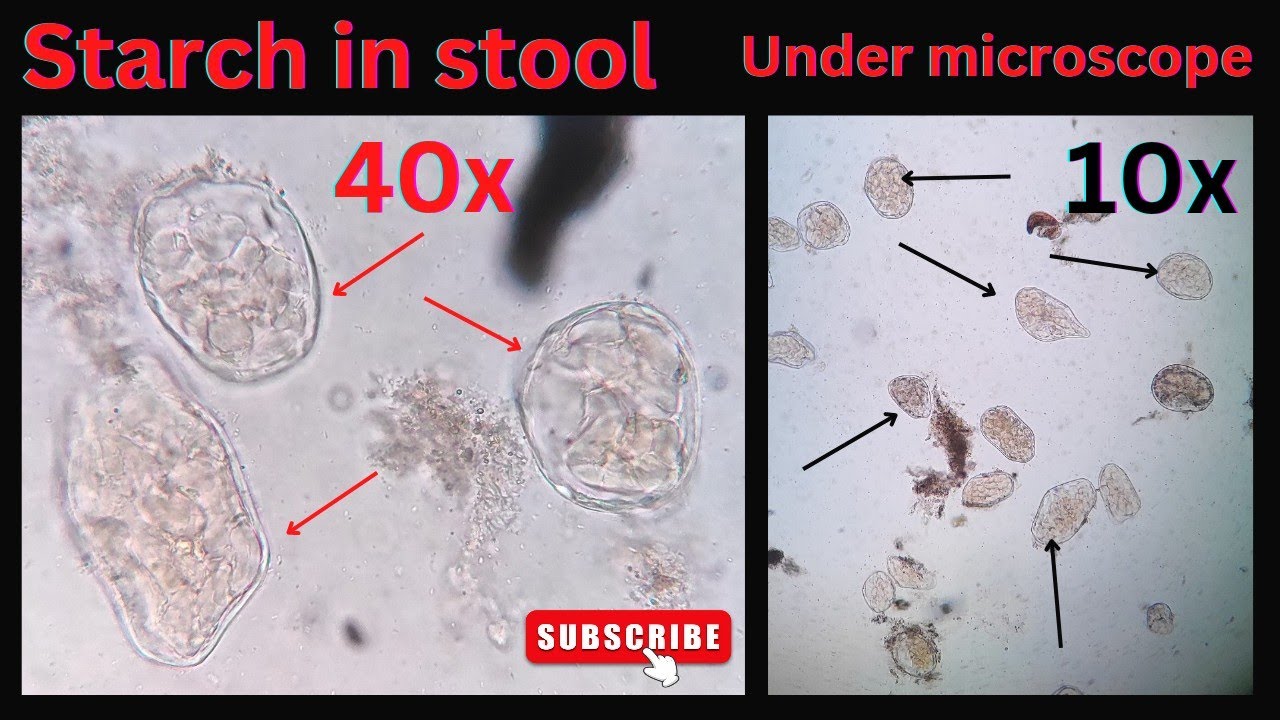The image displays two photographs of biological samples viewed under a microscope, presented side by side with a black border. A prominent header in bold red font reads "Starch in Stool Under Microscope." The photograph on the left highlights cell-like structures at 40X magnification, with three red arrows pointing to specific molecules, and the text "40X" in red. The photograph on the right shows similar structures at 10X magnification, with five black arrows indicating different molecules, and the text "10X" in black. The detailed magnified views provide a comparative perspective on the starch cells found in stool samples.